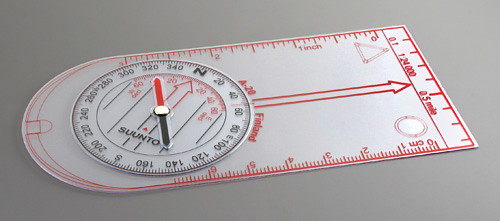A tightly focused, amateur photograph showcases a rather simplistic technical measuring device set against a grey, featureless background. The main object, which appears to be made of a thin, inexpensive white plastic, reveals an arched rectangular shape that occupies the entirety of the image.

This device is divided into three primary sections. Along one side of the arched rectangle are red markings indicating both inch and centimeter measurements, alongside another less clear scale, possibly denoting distances in miles up to 24,000 units. An arrow points to the only straight, short edge of the arched side.

Toward the left side of the device, there's a dial labeled "Suunto," suggesting it may be related to navigation. This dial, which seems capable of being manually rotated, features scales up to 340 degrees and an 'N' symbol, hinting at its possible use as a compass. Additionally, a black and red needle, mounted on a white circular piece with a white fastener, reinforces this theory. Despite the needle's presence, the device’s simplicity implies that it does not contain any digital or automated components, possibly requiring manual adjustment for directional readings.